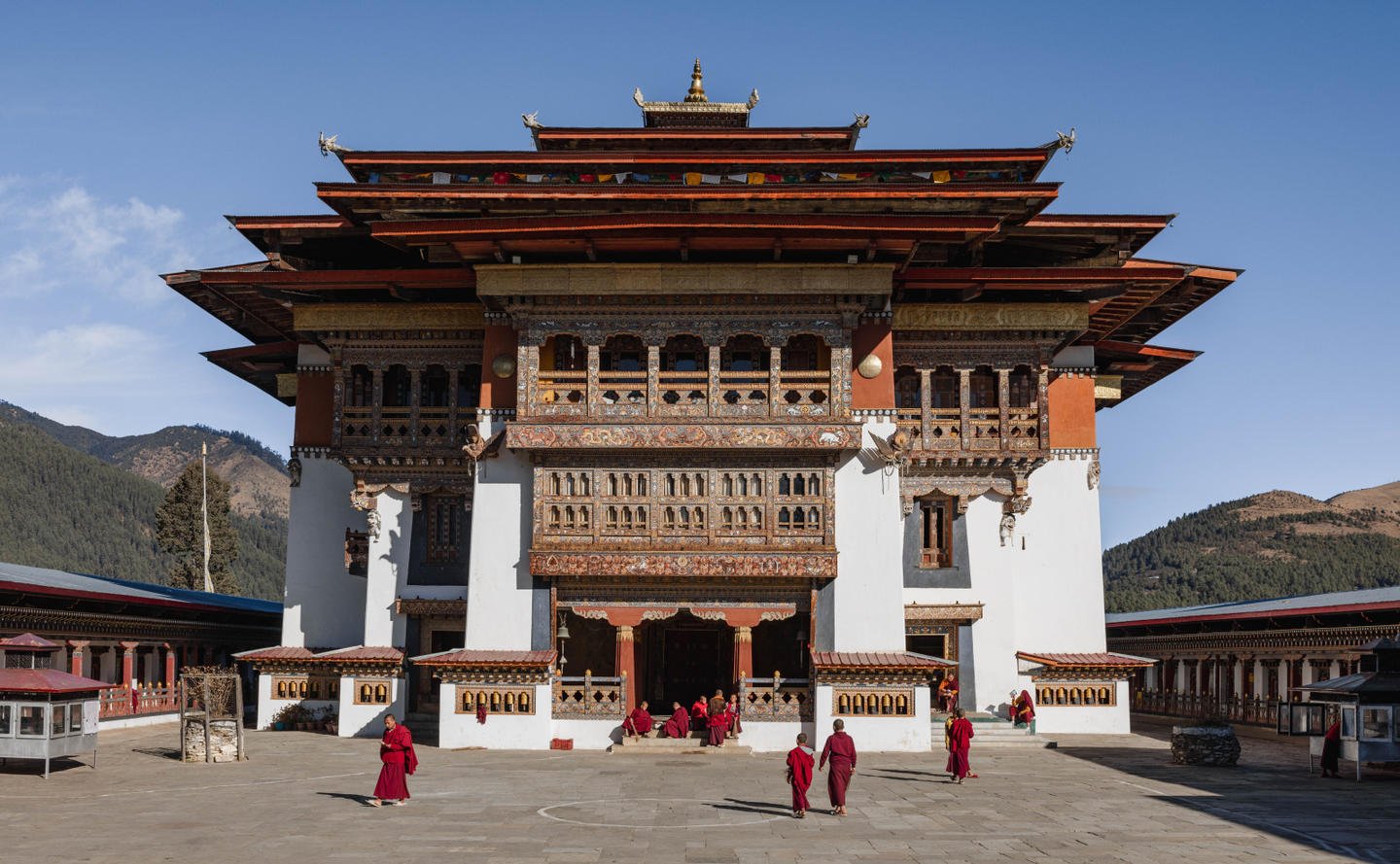The photograph captures a vibrant scene featuring a large, multi-storied Buddhist temple with intricate architecture dominated by white walls, red, gold, and brown decorative elements. The temple's upper level boasts arched windows beneath a pagoda-style roof adorned with golden bands. Central to the image, the temple is set against a backdrop of lush, green mountains under a bright blue sky with a few clouds. 

In the foreground, monks dressed in matching floor-length red robes are prominently positioned; several are seated on the temple's steps, while others walk towards the entrance and towards the lower left corner of the picture. Additionally, a couple of smaller buildings flanking the temple add to the complex's grandeur. The scene is imbued with a serene, religious ambiance hinting at the monks' involvement in prayer or meditation activities. The detailed beams and ornate features enhance the temple's majestic and sacred atmosphere.